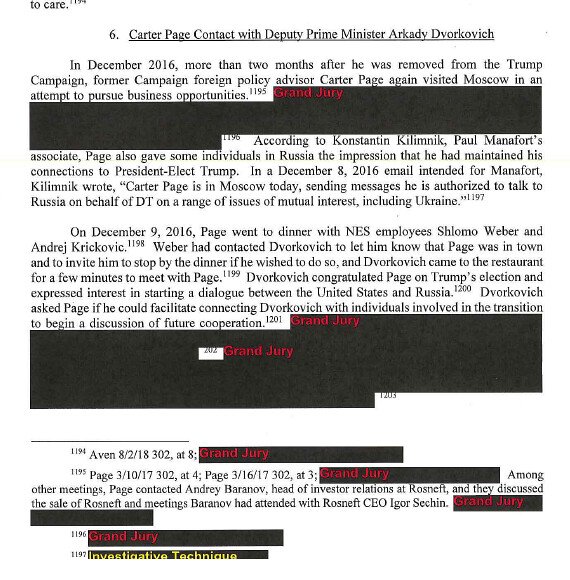The image depicts a redacted page from what appears to be a government report, likely from the Mueller investigation, based on its content and formatting. The page is titled "6. Carter Page Contact with Deputy Prime Minister Arkady Dvorkovich," and the title is underlined at the top. The text is predominantly in black Times New Roman font, interspersed with some phrases in red, notably the term "Grand Jury" linked to redacted segments.

The initial paragraph mentions that in December 2016, more than two months after being removed from the Trump campaign, former campaign foreign policy advisor Carter Page traveled to Moscow to explore business opportunities. Footnotes throughout the text cite sources, including one numbered 1195.

One section of the text has been blacked out, with the words "Grand Jury" in red over the redaction. The text that follows references an email dated December 8, 2016, from Konstantin Kilimnik to Paul Manafort, mentioning that Carter Page was in Moscow sending messages indicating he was authorized to communicate with Russian officials on behalf of Donald Trump.

On December 9, 2016, Page had dinner with NES employees Shlomo Weber and Andrei Krykovich. Weber had informed Dvorkovich about Page's presence in Moscow and invited him to join the dinner. Dvorkovich briefly attended, congratulated Page on Trump's electoral victory, and expressed interest in initiating dialogue between Russia and the United States. He also inquired if Page could help facilitate connections with individuals involved in the U.S. presidential transition to discuss future cooperation.

The latter part of the text is significantly redacted, again marked by the term "Grand Jury" in red, obscuring substantial portions of the narrative up to the document's footnotes at the bottom.

Overall, the image provides detailed insights into Carter Page's interactions with Russian officials and indicates ongoing investigations relevant to these events.